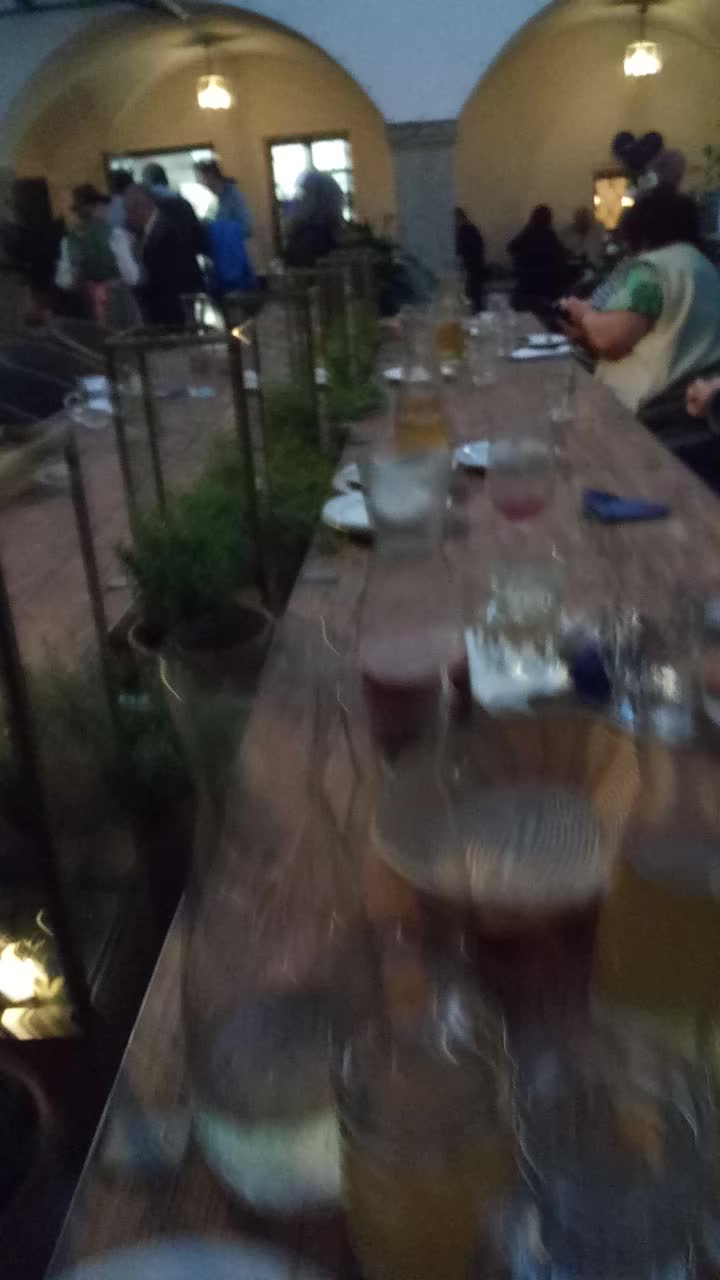This vertically cropped, blurry color photograph captures a lively restaurant gathering. A long buffet table extends diagonally from the bottom left to the upper right quadrant. Beneath the table, a row of potted plants adds a touch of greenery. The table is adorned with an assortment of glasses filled with various colored liquids and small saucer plates, indicating a vibrant selection of refreshments. In the background, balloons decorate a wall, contributing to the festive atmosphere. Two architectural arches frame the scene, adding to the restaurant's charm. Near the far end of the table, a woman wearing a white vest is seen leaning over, possibly arranging items or serving guests. A crowd of attendees congregates in the back left portion, socializing and enjoying the event. Despite the image being blurry and out of focus, the convivial spirit of the gathering is evident.